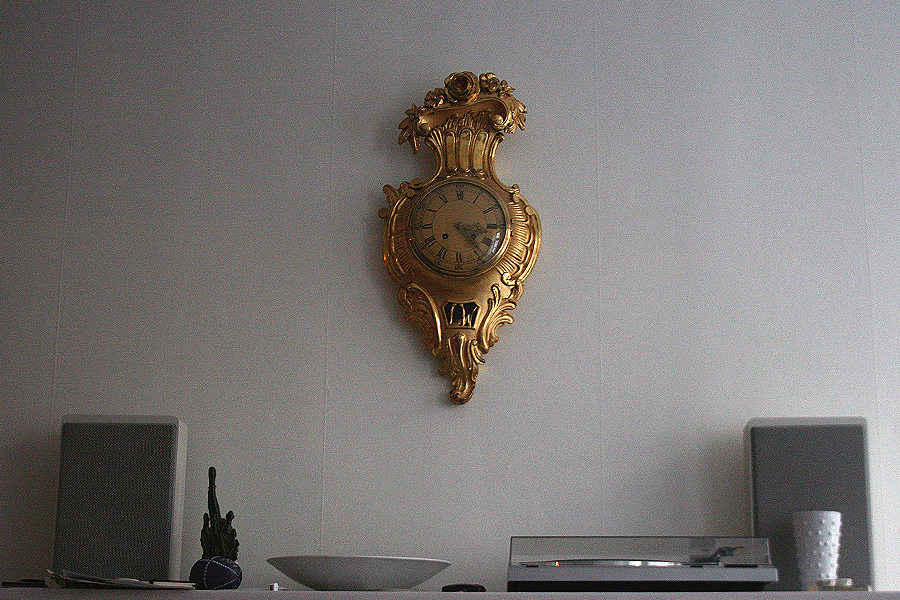The image depicts a well-furnished living room adorned with a striking Rococo-style gold clock mounted on a gray wall. The clock features an intricately designed face with Roman numerals and black hands, showing a time around 3:18 to 3:25. The clock's ornate structure includes a bouquet-like top and a scone-shaped bottom, exuding an antique aesthetic.

Below the clock, there's a flat, gray surface, possibly a TV stand or console, holding a variety of objects. A record player sits in the center, flanked by two speakers. In front of the right speaker, there's a distinctive white vase with a knobby, textured surface. To the left of the record player, an array of items includes a large white ceramic bowl, a small dark flat object, an intricate ornament, and a fabric egg. Additionally, there are some papers placed in front of the left-hand speaker, adding to the lived-in feel of the room. The overall scene combines modern elements with classical ornamentation, creating a unique and detailed living space.